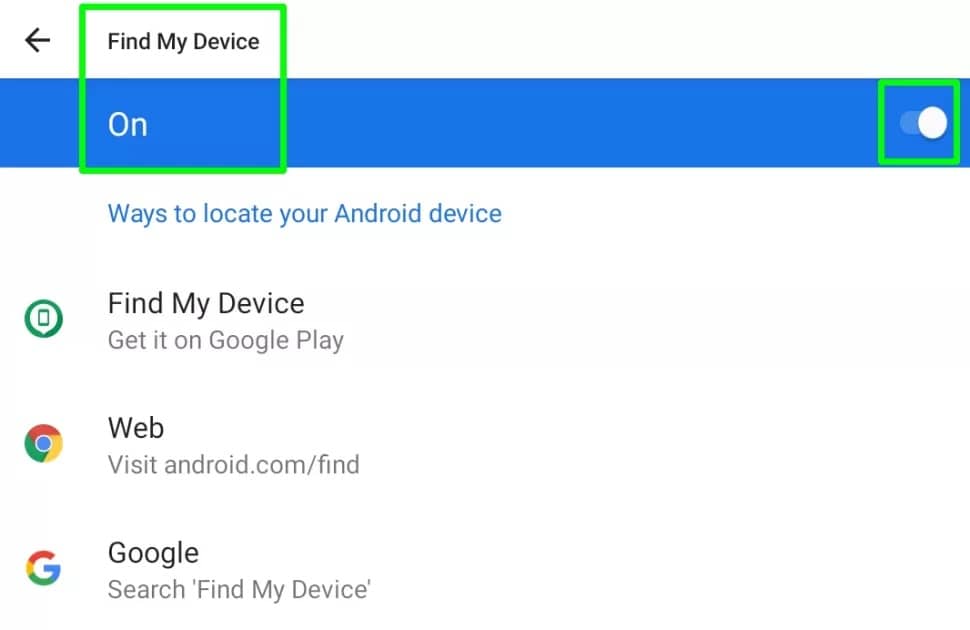The image displays the "Find My Device" settings section on a smartphone. At the top left corner, there's a back button denoted by a left-facing arrow. Below it, a green box highlights the "Find My Device" option, indicating that it is enabled. To the far right of this option, a green toggle button confirms its active status. 

Underneath the green box, blue text reads "Ways to locate your Android device." Listed vertically, there are several options:
1. A smartphone icon followed by "Find My Device" and "Get it on Google Play."
2. A Google logo with the text "Web" and the URL "visitandroid.com/find."
3. Another Google logo with the text "Google" and the instruction "Search 'find my device'."

The webpage provides multiple methods to locate an Android device, with the "Find My Device" feature currently toggled on.